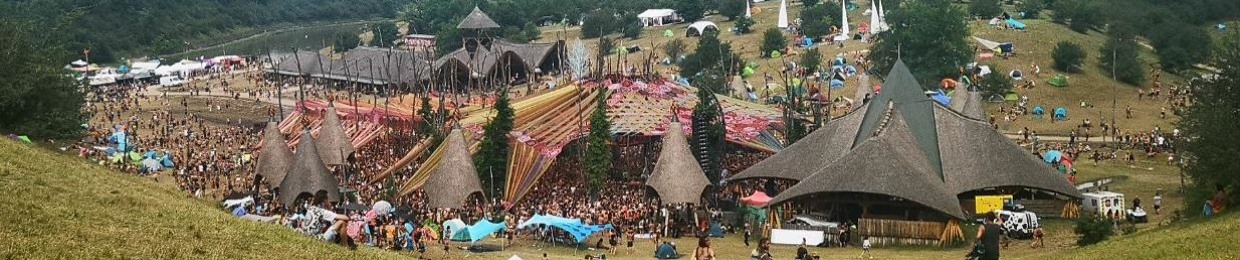This detailed panoramic photograph, likely taken from an elevated vantage point such as a drone or an airplane, captures a lively festival set within a picturesque valley surrounded by rolling hills and tall evergreen trees. In the foreground, at the base of a grassy hill dotted with coniferous trees, clusters of cone-shaped tents and larger makeshift structures are arranged, hinting at a medieval cosplay theme. At the center of the image, under the shelter of a massive fabric tent, a bustling crowd gathers, suggesting a grand central venue that can accommodate hundreds, if not thousands. To the left, there are permanent buildings with gray and white exteriors, further adding to the venue's extensive setup. The photograph, with its wide-angle and horizontal orientation, encapsulates a vibrant scene of people, tents, and canopies all set in a scenic valley amidst a verdant, hilly landscape.